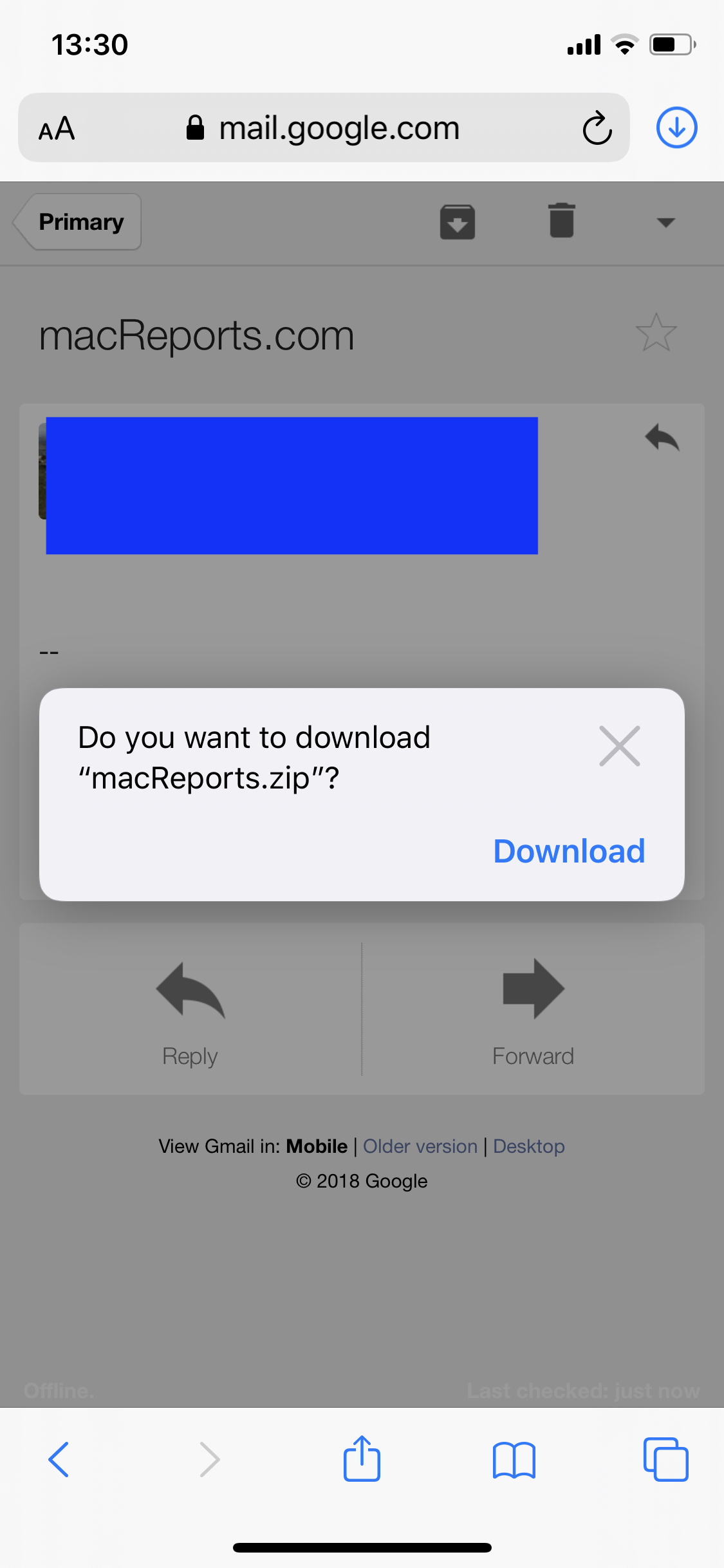The image depicts a smartphone screen displaying an email interface with intricate details:

At the very top, the screen shows the time along with various icons including Wi-Fi signal strength, battery percentage, and cellular signal indicator. The browser's URL bar features a padlock icon, the address "mel.google.com," and a circular blue download button with a downward-pointing arrow.

The main content of the screen is an email from "macreports.com," characterized by a blue header bar and a predominantly white and gray background. There is a prominent popup message asking, "Do you want to download macreports.zip," accompanied by a blue download button and a gray 'X' for closing the popup.

Within the email's interface, there are several interactive elements: a reply button marked with a leftward-facing arrow and a forward button denoted by a rightward-facing arrow. Additionally, near the bottom of the screen, there's an option to "View Gmail in mobile, older version, or desktop," followed by the note "2018 Google."

At the footer of the screen, there are several functional buttons, including a blue back arrow, a gray forward arrow, an upward-facing arrow for sharing, a bookmarks tab represented by an open book icon, and two overlapping blue squares indicating an option to manage open tabs.